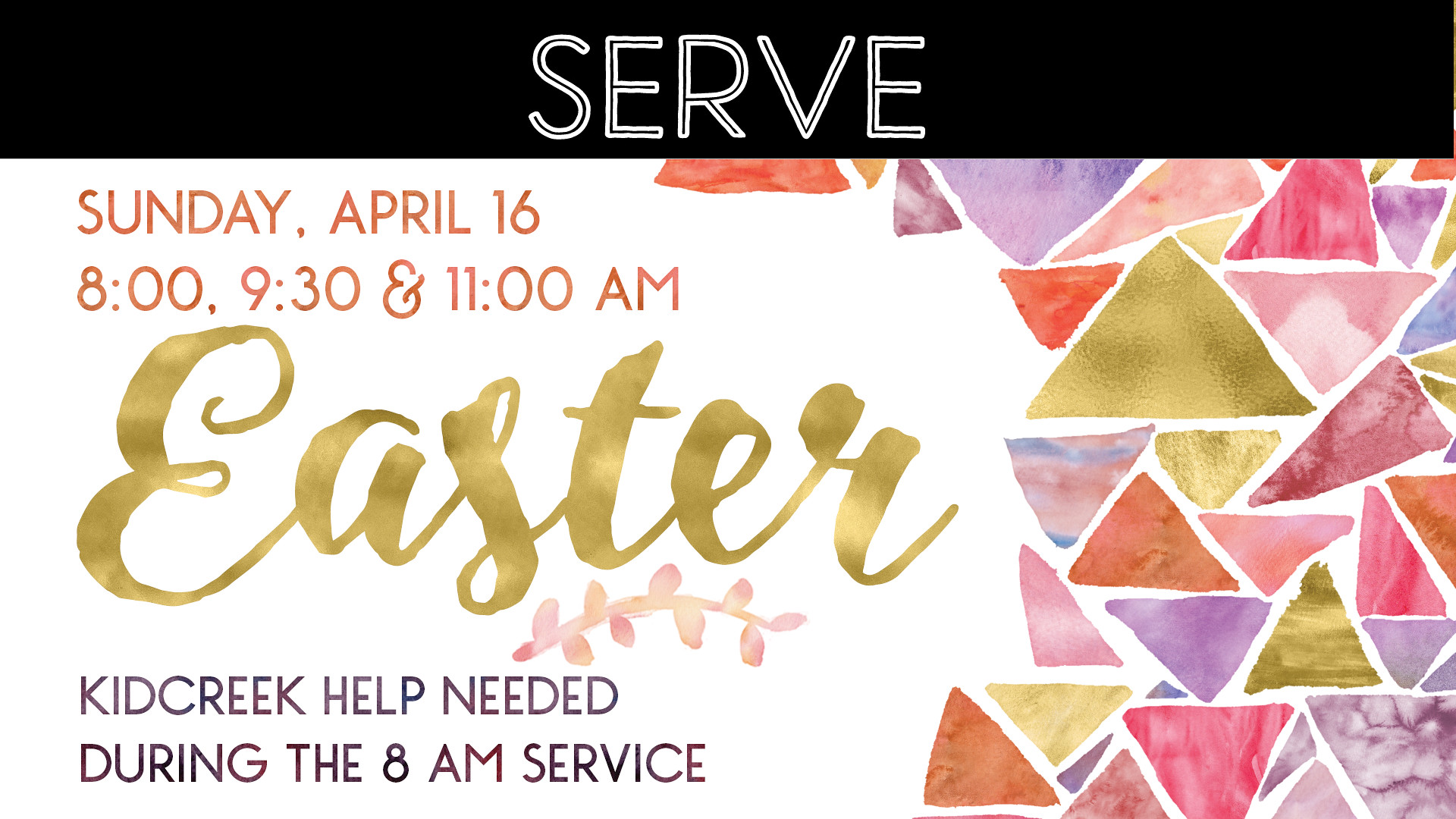This image serves as an advertisement for a church's Easter service, designed as an infographic suited for a website or social media. At the top, a black bar displays the word "SERVE" in large white letters. Below, the primary background is white adorned with abstract, pastel-colored watercolor triangles in shades of gold, pink, orange, and purple along the right-hand side. Beneath the "SERVE" text, it announces the date and times for the Easter service: Sunday, April 16th, with services at 8:00 a.m., 9:30 a.m., and 11:00 a.m. Centered and prominent in large gold cursive text is the word "EASTER," accompanied by a delicate pink and peach floral design underneath. At the bottom, it conveys an additional message, "Kid Creek help needed during the 8 a.m. service." This landscape-oriented invitation emphasizes the need for volunteers and provides detailed information about the Easter service timings, complemented by a visually appealing geometric pattern.